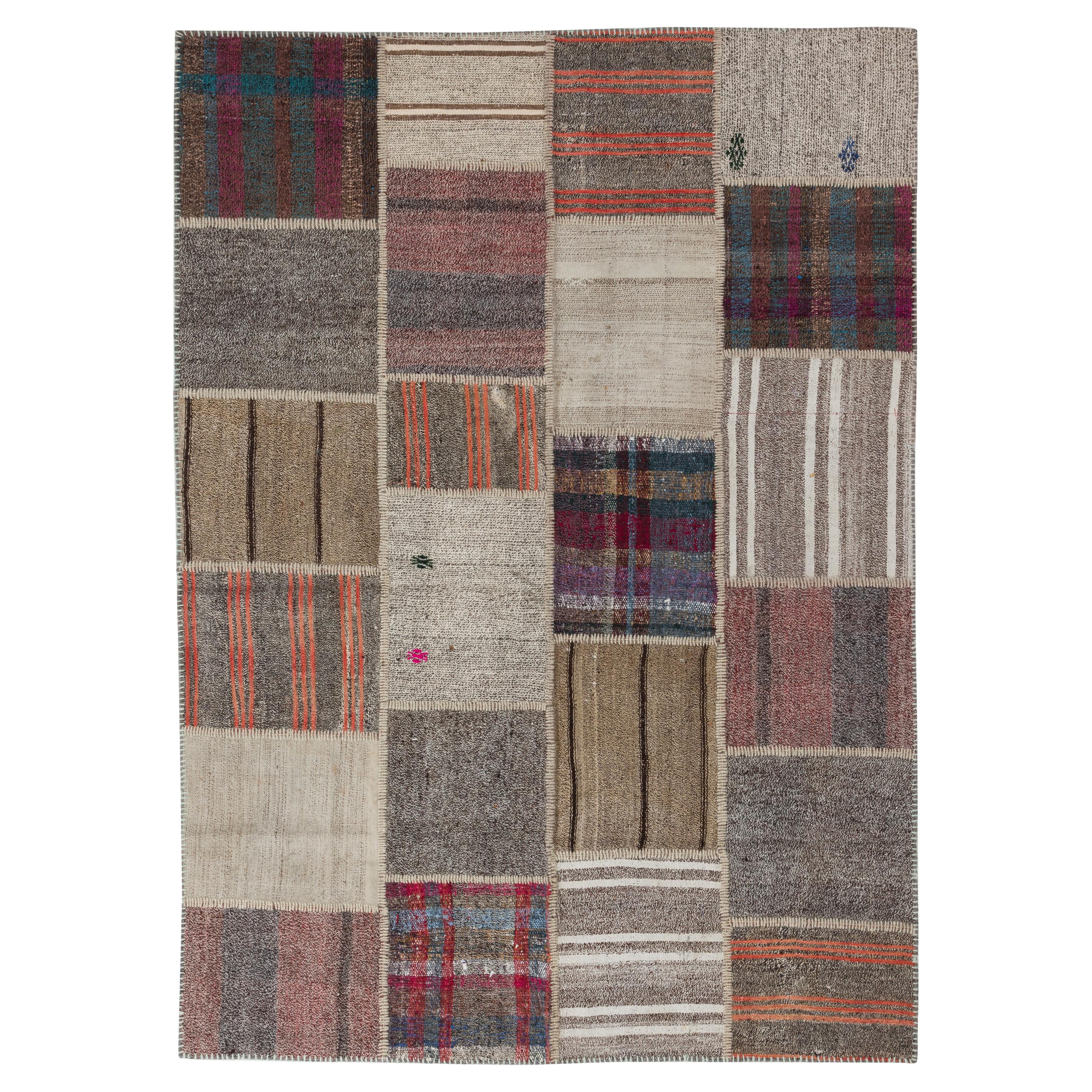This photograph showcases a patchwork quilt composed of numerous squares of fabric, each with varying colors and textures. The quilt features over two dozen visible squares, most of which exhibit either stripes or plaid patterns. The primary color palette is composed of earthy and neutral tones, with an abundance of browns, tans, and light browns, punctuated by occasional whites. Some squares stand out with additional colors, such as a bottom right corner piece adorned with orange stripes and a top left corner square that incorporates more vibrant reds and blues. Despite these bursts of color, the overall aesthetic of the quilt remains subdued and cohesive, aiming for an earthy, understated look. The squares themselves vary in size and are sewn together with a grayish-brown basting border, enhancing the quilt's patchwork charm.